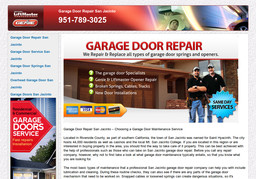The website header features a gradient of red shades with a blurry section in the upper left corner, possibly containing the company's name, though it is not legible. Adjacent to this, a clear white phone number is visible: 951-789-3025. The left side again presents unclear blue text. On the lower part, an image shows a house roof design with a red pentagon enclosing the text "Garage Door Service" in white. Above this, black text potentially states "Residential or Commercial," while yellow text of unknown content lies beneath it. 

The background predominantly consists of an off-white hue, with bold red text stating "Garage Door Repair" followed by illegible black text. The image also includes two men who appear to be employees, dressed in company shirts and blue jeans, within a uniquely-shaped blue circle that contains the black text: "Read Our Services." Notably, logos for payment methods such as American Express, MasterCard, and Discover are visible, indicating the accepted cards. The bottom section of the website has a large amount of black text, likely providing further details about the company and their services, although this text remains too blurry to discern.